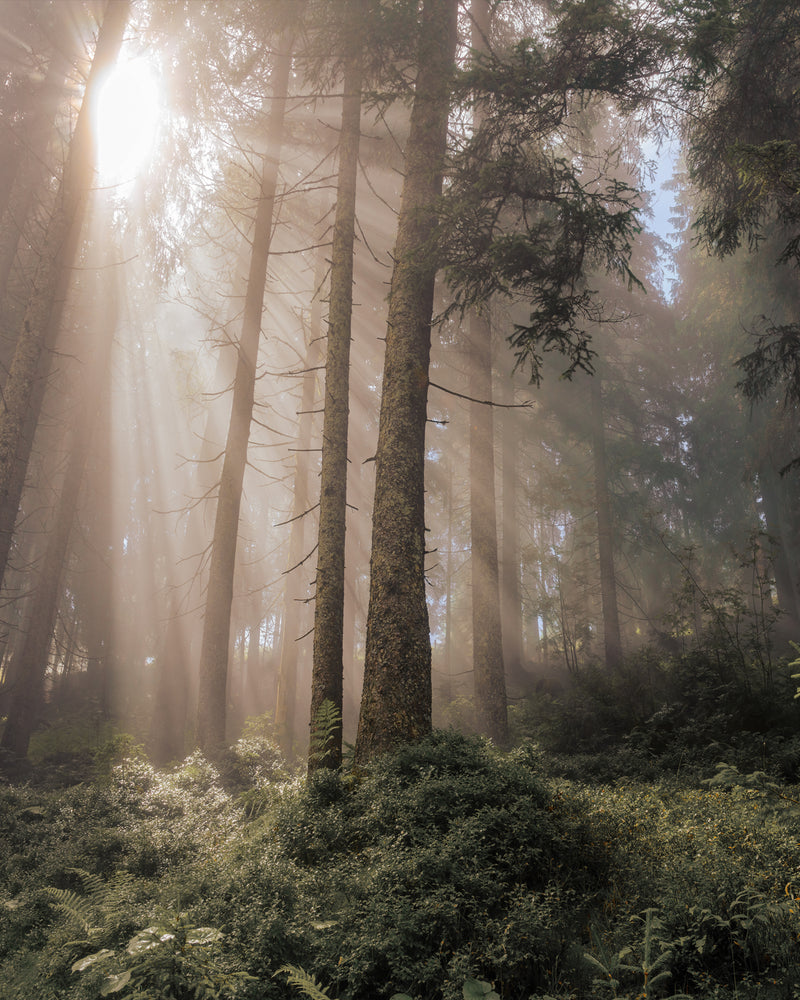This forest scene, depicted in a tall, portrait-oriented photograph, captures the serene beauty of a lush, steep hillside. The lower portion, comprising roughly 20% of the image, is a verdant carpet of ferns and a variety of green vegetation. At the center stand two prominent tree trunks, their numerous branches climbing upwards before bursting into a canopy of green leaves at the top. Surrounding these central trees is an array of faint, nearly blurry tree trunks, adding depth to the background and showcasing a dense, forested area. 

Hints of blue sky peek through the canopy, predominantly visible in the upper right. The upper left corner of the image is graced by an oval-shaped white spot representing the sun. Its rays stream through the branches and leaves, casting a warm, yellow-white light that illuminates the foliage and forest floor below. Adding to the mystical ambiance, the interplay of sunlight and morning fog creates a misty glow, enhancing the tranquil and enchanted feel of this evergreen forest.